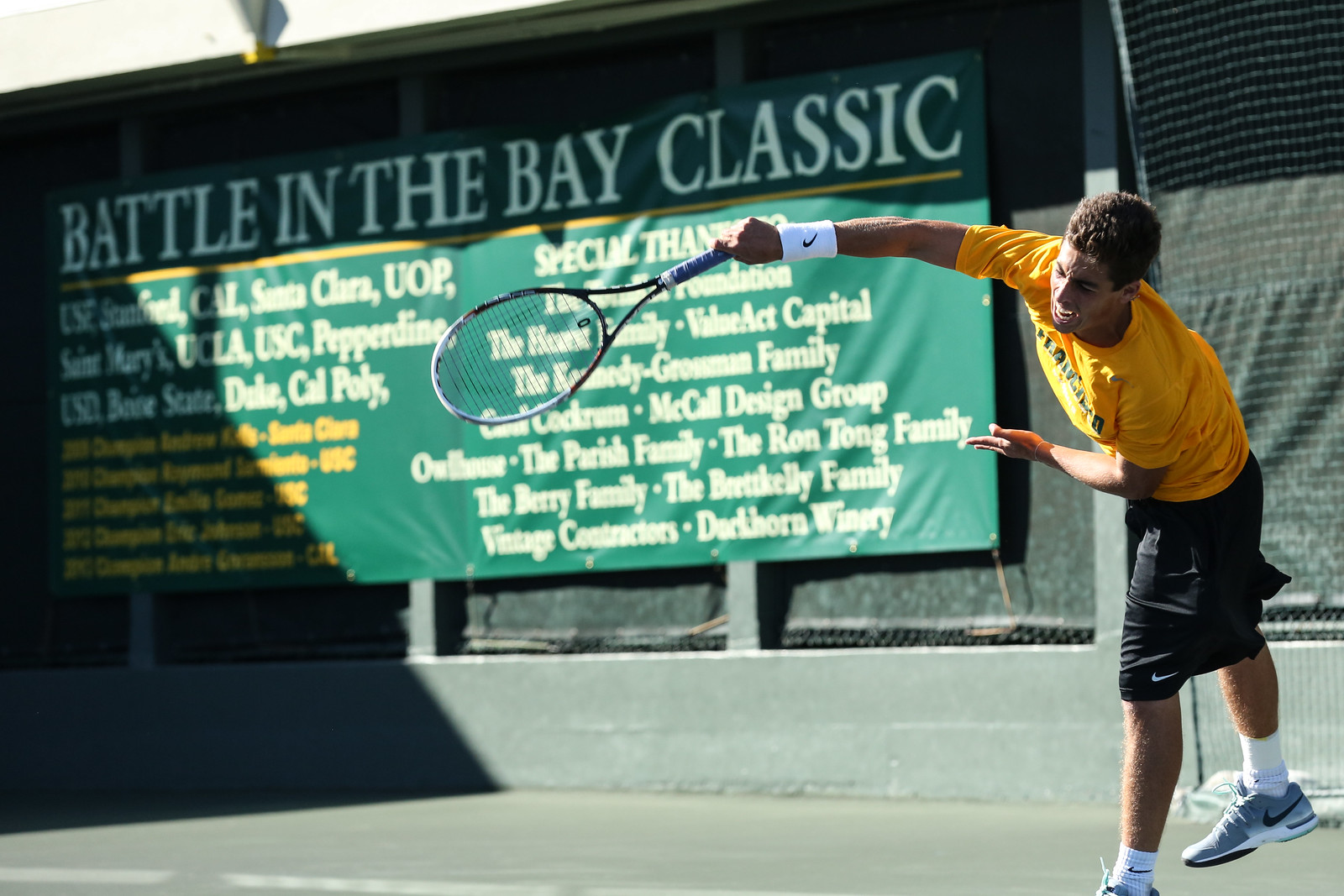This outdoor daytime photograph captures a dynamic moment of a tennis player mid-action. The man, with light brown skin and dark brown hair featuring some blonde highlights, is intensely focused as he plays on a green tennis court. He is wearing a short-sleeved orange t-shirt, black Nike shorts, gray Nike sneakers, white Nike socks, and a white Nike wristband on his right wrist. His athletic stance, bent forward at the waist, shows his right arm extended and holding a tennis racket high, suggesting he is in the follow-through of a powerful shot. His left arm is bent and tucked in, while his right foot is lifted behind him, illustrating his balance and agility. The background features gray concrete fencing with mesh netting adorned by a large green banner bearing the bold white letters: "Battle in the Bay Classic." Although some text on the banner is blurry, it details the various cities hosting the classic, likely colleges, and expresses special thanks to families, individuals, design groups, and foundations.